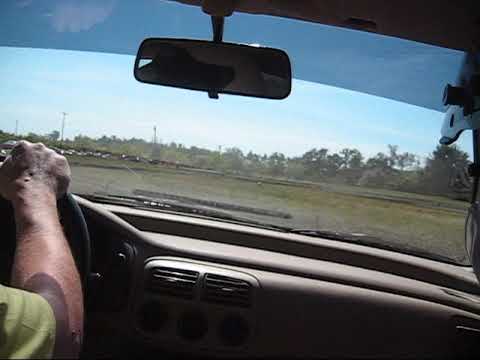The image captures the perspective from inside a car, seemingly from the back seat, looking forward through the windshield. The foreground prominently features the interior of the vehicle, including part of the steering wheel and dashboard, which has various controls and AC vents. The dash is partially illuminated by sunlight, with the area below being shadowy and indistinct. Notably, the right side of the image shows a driver wearing a white helmet, partially obscuring the view of the steering wheel.

The middle section of the image encompasses the rearview mirror, which reflects a string of small flags. Above the mirror stretches the sunshade at the top of the windshield. Beyond the car's interior, the windshield offers a view of an open, grassy area containing a man standing slightly right of center. In the far distance, there are trees under a cloudy, blue sky. Additional details include what appears to be an electric pole behind the man and a gravel drive or dirt path extending from the front of the car to the grassy area, bordered by a bit of a curb and grassy mounds. To the left, something is on the back driver’s side of the car, but its exact nature is obscured by darkness.